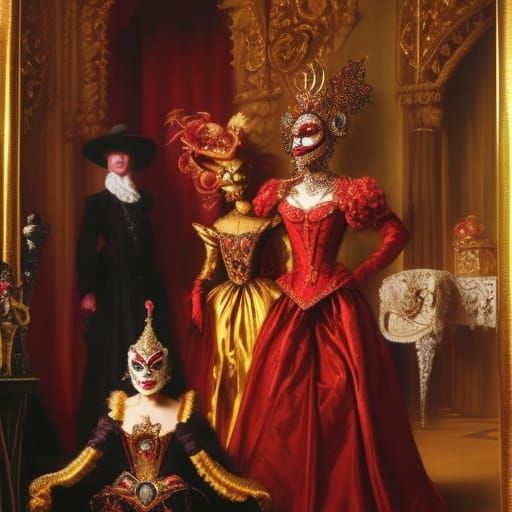The image depicts an elaborate, AI-generated masquerade scene that emulates the style of a 17th-century painting. The focal point is on two women adorned in opulent ball gowns and intricate masks. The woman on the left is seated, wearing a red dress with large shoulder pads and a distinct mask featuring white and red accents. The standing woman beside her is dressed in a purple and yellow gown also accompanied by an ornate mask. The backdrop is a lavish room with gilded cornices and red drapery, and there is a sense of overwhelming opulence throughout. An ornate piano is visible in the background, along with a mannequin or perhaps a figure dressed in a black Three Musketeer-style outfit. Additionally, there is another figure or mannequin in a golden, butterfly-like dress and a towering wig, as well as a man in distinct attire with a scarf and hat, adding to the enigmatic and peculiar atmosphere of the scene.